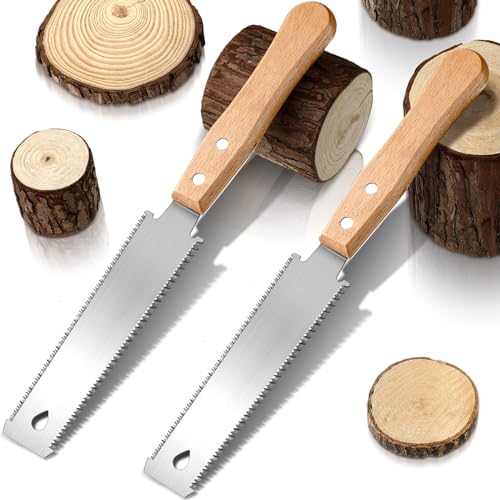The image displays two small handheld woodworking saws resting on several cut pieces of log segments, on what appears to be a white background. Each saw features a wooden handle akin to those found on steak knives, with visible grain patterns, and double-sided serrated silver blades. The saws, angled downwards with their blades touching the surface, are identical and include a chisel-like tip and a metal feature at the bottom, potentially for nail pulling or detailed cutting. Surrounding the saws are multiple log sections of varying sizes, some standing upright and others lying on their sides, displaying the contrasting brown bark and blonde wood interior. One log segment appears cut in such a way that slices have been sawn off, indicating the fine, precise work these saws are designed for.